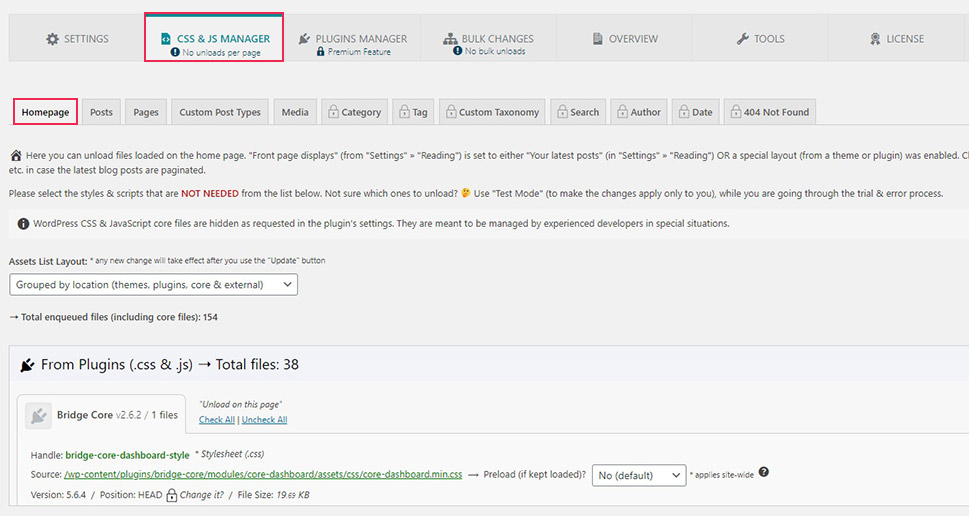The image depicts a settings page on a slightly gray background, with a slightly darker gray border surrounding the settings title area. At the top, a bordered section displays the word "Settings." Beside it, in a red rectangular box, is labeled "CSS and JS Manager - No unloads per page." Continuing, there are several options listed: "Plugins Manager (Premium feature)," "Bulk Changes," "No Bulk Unloads," "Overview," "Tools," and "License."

Below this section, there is another row of categories outlined in red with labels such as "Home Page," "Post Pages," "Custom Post Types," "Media," "Category Tag," "Custom Taxonomy," "Search," "Author," "Date," and "404 Not Found." 

The description indicates that on this page, you can manage the unloading of files loaded on the front page. It mentions that the front page displays settings equivalent to either your latest posts or a specific layout enabled by a theme or plugin. The image implies that the latest blog posts are paginated, and users can select the styles and scripts that are not needed from the list.

It provides a note suggesting the use of Test Mode to ensure changes only apply to the user during the trial and error process. Additionally, it mentions that WordPress core files related to CSS and JavaScript are hidden, as requested in the plugin settings, meant for experienced developers in special situations. 

Information about asset management indicates that any new changes will take effect after using the update button. The items are grouped by location: themes, plugins, cores, and external. The total enqueued files include 154 from plugins (.css and .js) and a detailed breakdown showing 38 files related to BridgeCore Dashboard styles, their paths, and settings such as "mincss preload" and "No by default."